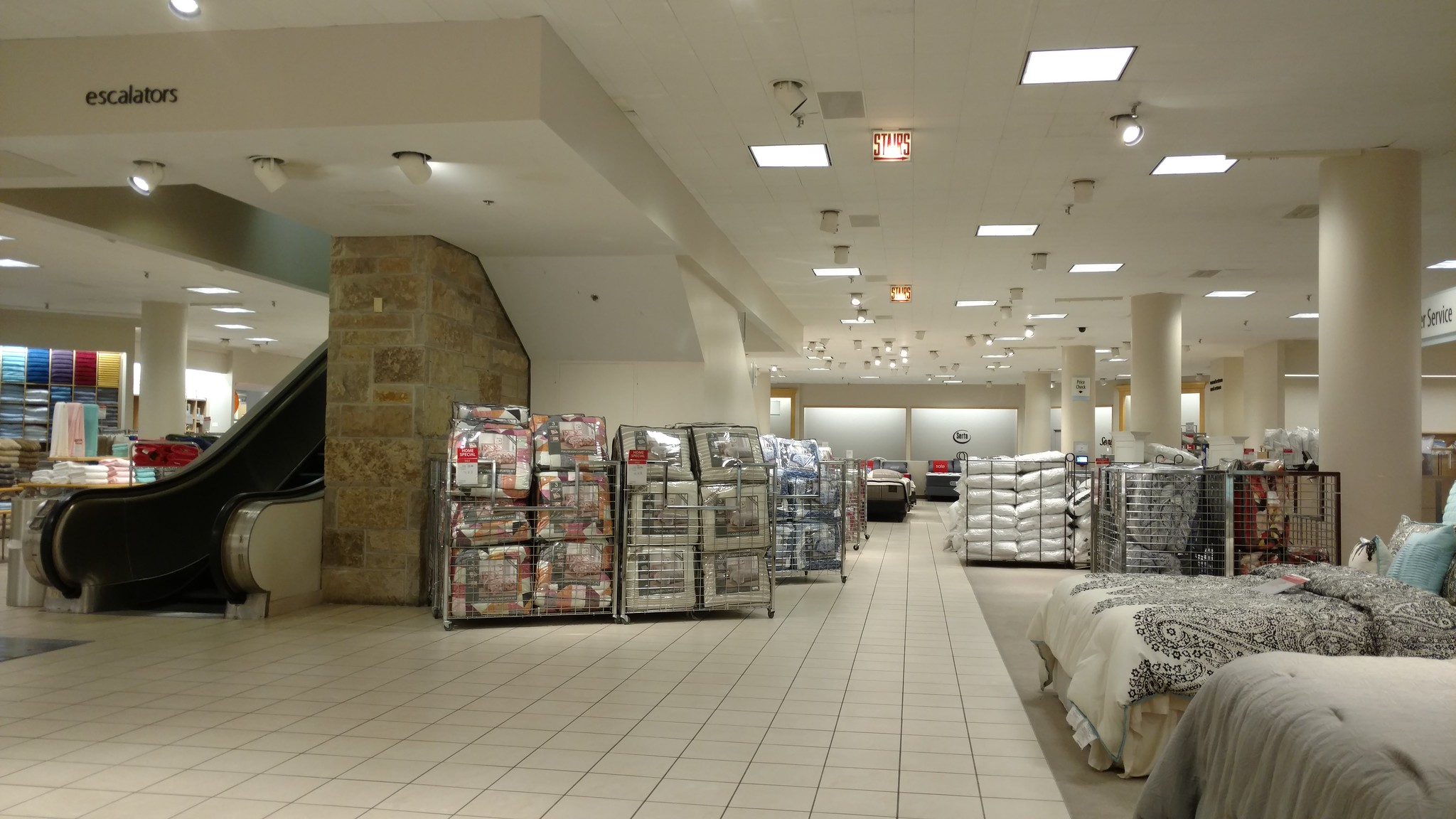This color photograph captures the interior of a large department store, specifically within the linen department. The scene features an extensive white or off-white 12-inch tile floor with light gray grout, which transitions to a carpeted area on the left. Running down the right side are cylindrical white columns stretching into the distance. Toward the right, several beds are displayed, adorned with a variety of comforters and fabrics in colors such as gray, brown, black and white, and blue. Nearer the foreground and further back, bins and stacks of pillows can be seen, along with comforters in plastic bags.

To the left of the image, a black escalator ascends beside a rustic brick wall, with a sign overhead indicating its presence with black letters spelling "escalators." Vividly colored towels, including shades of red, yellow, green, purple, turquoise, and white, are displayed above the escalator. The white ceiling is outfitted with both fluorescent lighting and spotlights to highlight various displays. Additional ceiling features include vents, sprinklers, and lit signs that read "stairs" in red on a white background. The image stretches far back, revealing the depth and vastness of the store's interior.